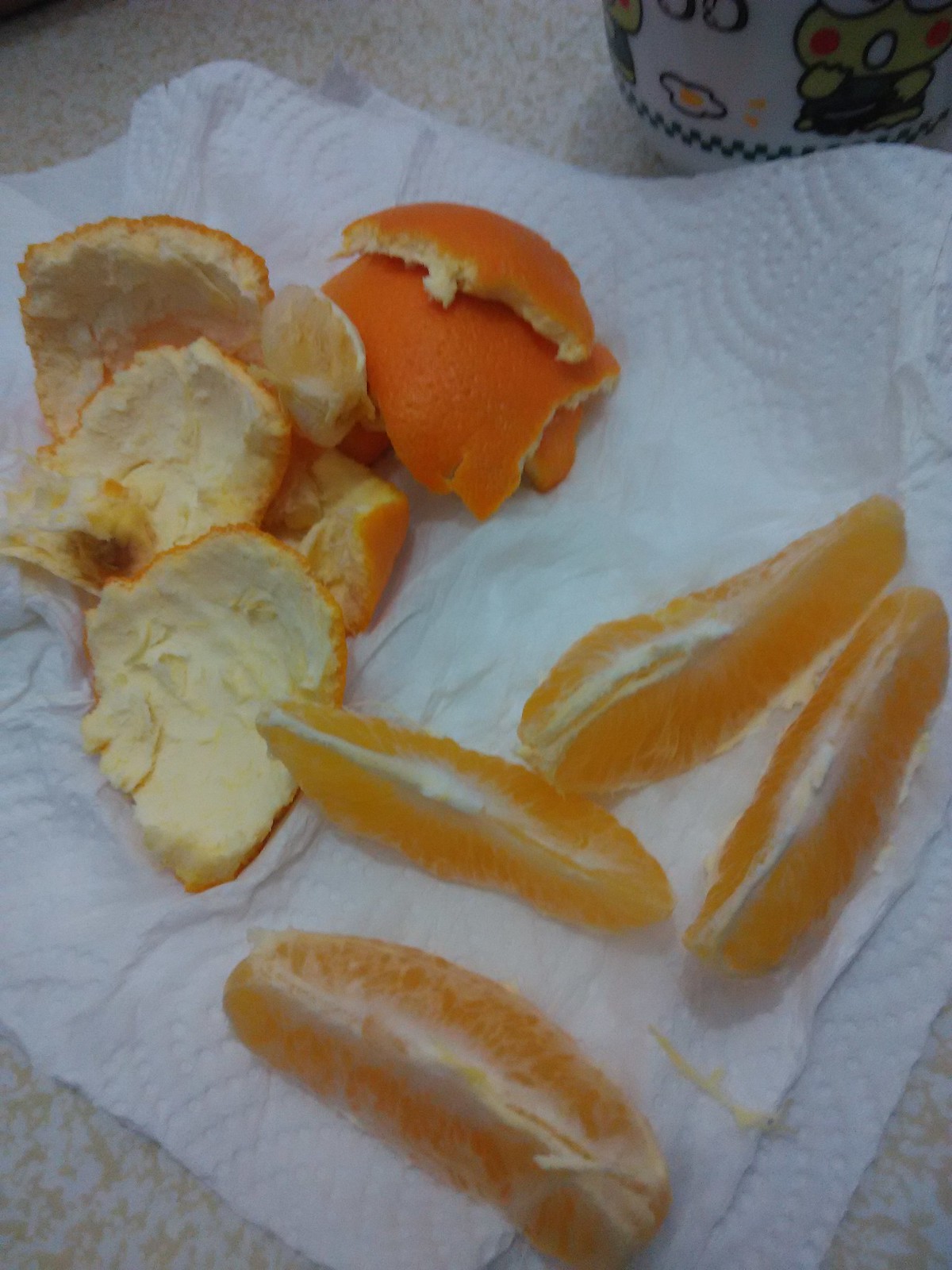A detailed photograph depicts a tabletop covered in a white Formica-style surface with small brown flecks. Central to the image is a diagonally positioned white paper napkin, showing noticeable creases and folds, suggesting it was previously crumpled. On the left side of the napkin, there are approximately eight pieces of discarded orange peel. To the right, the napkin holds four neatly arranged orange segments, with some of the white, stringy fiber from the peel visible between them. Just touching the top right corner of the napkin is a small, character-designed white cup, reminiscent of a child’s plastic drinking vessel, featuring colorful, anime-style cartoon figures. The table surface is visible in the bottom corners and edges of the image, framing the napkin and its contents.